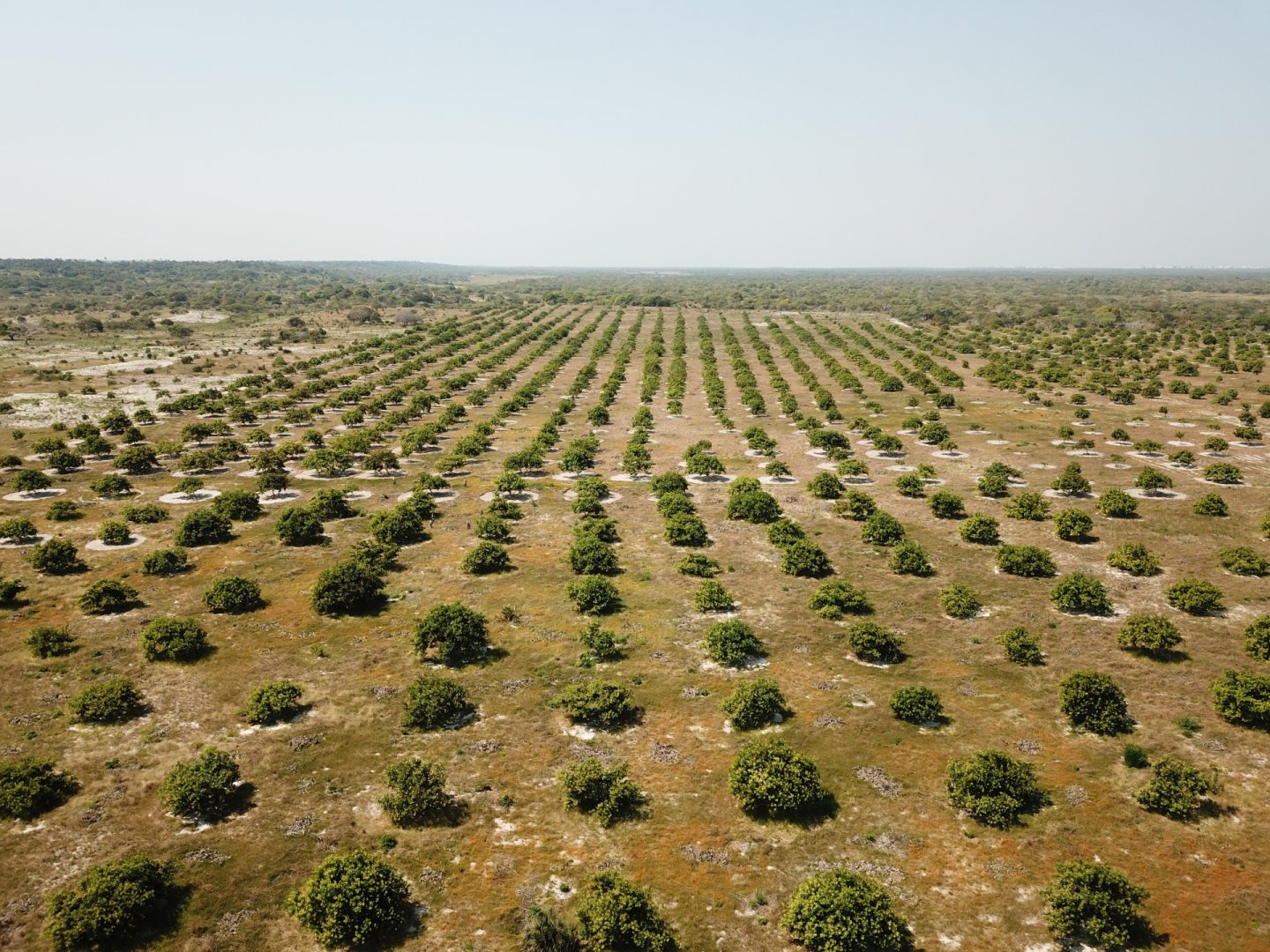The image depicts an expansive outdoor scene featuring a large, evenly spaced orchard or tree farm planted in long, meticulous rows. The trees, which are dark green but not vibrant, appear round-topped and are in various stages of growth, with some sections showing younger, smaller trees. The field stretches from the foreground towards a distant mountainous hill area, under an overcast sky that is a mix of gray and blue hues. The ground in the field is mostly dry with short, brownish-gray grass, dotted with small white circles under the trees, likely indicating some form of irrigation or protective measures. Sporadically, there are gaps where some trees have died and need replanting. Beyond the orchard, the landscape transitions into a greener, forested area with what appears to be a lake visible in one direction, adding depth to the serene yet methodical agricultural setting.